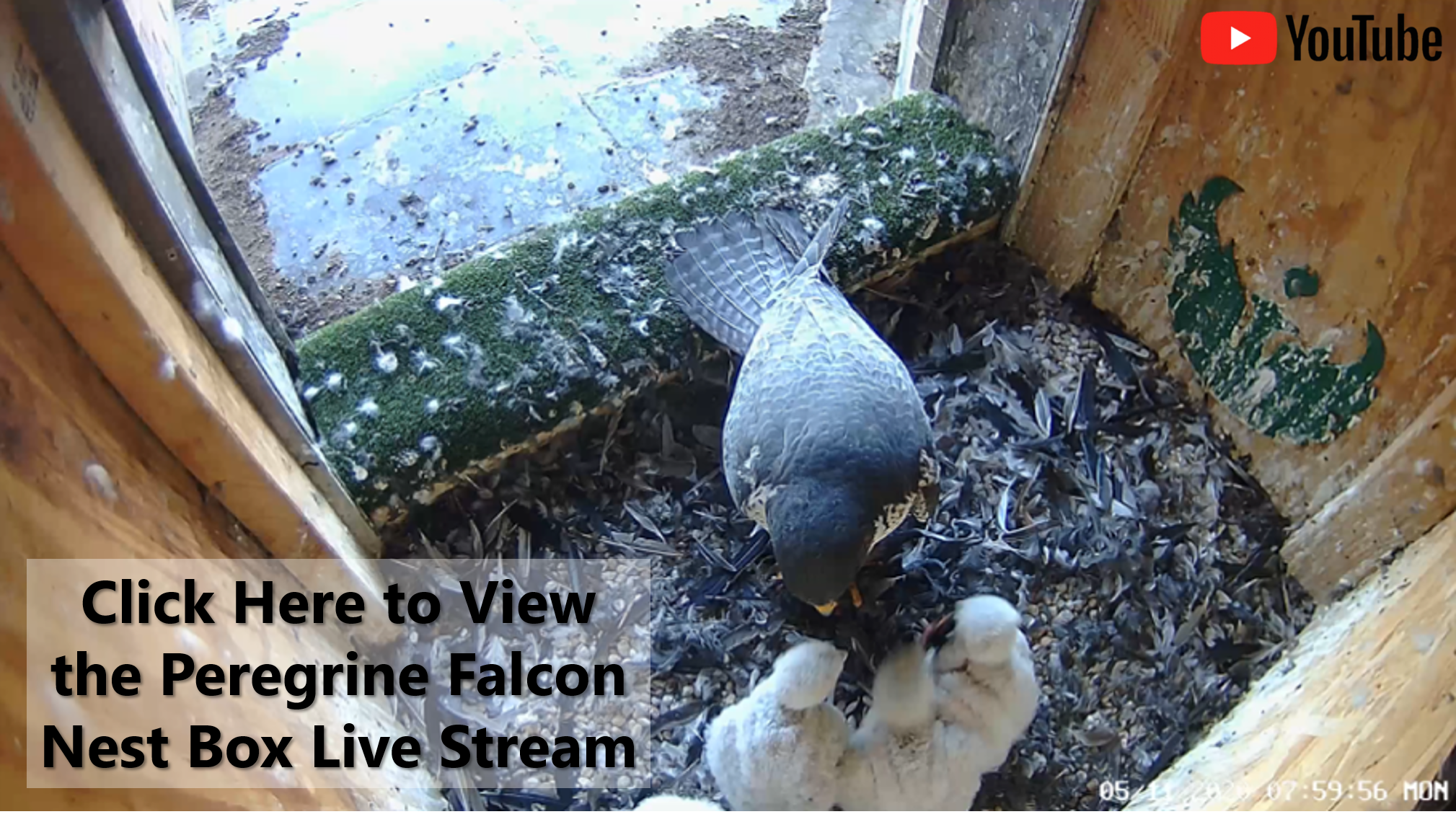The image is a screenshot of a YouTube video thumbnail featuring the inside of a peregrine falcon nest box. In the upper right corner of the image, the YouTube logo is clearly visible. Centered in the frame is an adult peregrine falcon, black in color, standing over three fluffy, white baby falcons that resemble large cotton balls. The nest box itself is constructed from wood, with sides forming a wooden enclosure. The ground is covered with feathers and appears greyish, with stones and scattered leaves. There are also some green drawings visible on one side of the wooden enclosure. In the bottom left corner of the image, a text overlay reads, "Click here to view the peregrine falcon nest box live stream.”